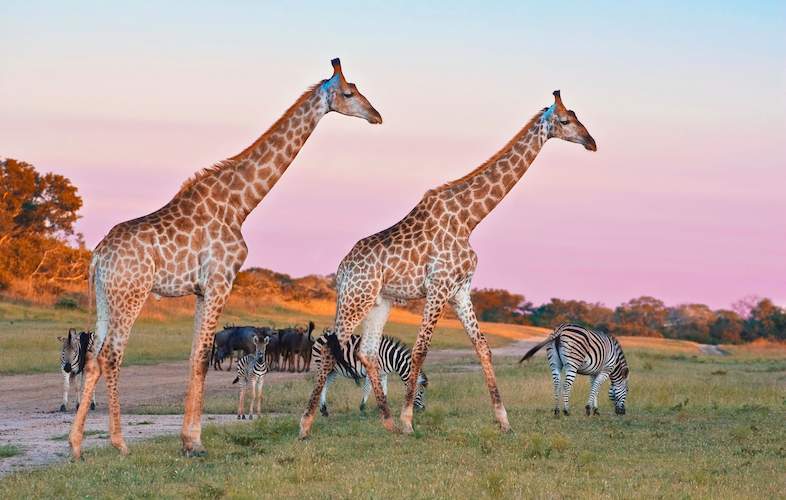In this stunning wildlife photograph taken during sunset, two adult giraffes with distinct blue tags on their ears are seen walking along a dirt road. The sunset casts an enchanting orange glow across the landscape, illuminating the background trees with a golden hue and creating a sky painted in shades of pink and light blue. Alongside the giraffes, four juvenile zebras are visible, grazing and wandering on the grassy areas adjacent to the road. Other animals, including what appear to be black buffaloes, can be observed in the distant background, adding depth to this picturesque scene that epitomizes coexistence in nature. The overall ambiance suggests the skillful work of a wildlife photographer capturing the serene beauty and harmony of the wilderness at twilight.